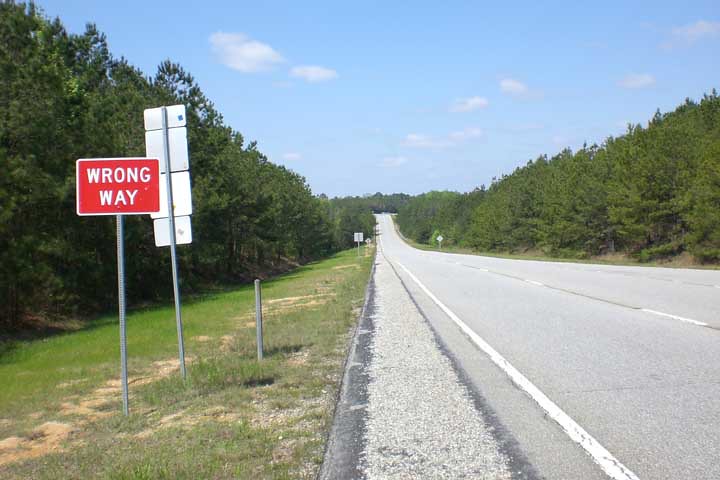The image depicts a long, deserted two-lane highway, likely part of a four-lane parkway, bordered by grass and trees on each side. The asphalt road is pale gray with white lines, featuring a solid white line on the left demarcating the emergency lane and a dotted white line separating the two lanes heading away from the viewer. Prominently in the foreground on the left side, there's a red "WRONG WAY" sign with white lettering, mounted on a gray metal pole. Behind this, closer to the viewer, are several signs with their backs visible, supported by poles but unreadable from this angle. The shoulder of the highway is sandy with patches of weedy, unmanicured grass, and immediately adjacent is a grassy verge leading into a dense border of trees that are possibly a mix of deciduous and evergreen species. The sky is a vivid blue with scattered puffy white clouds, indicating a pleasant, sunny day with no visible traffic or human activity on the road stretching into the distance.